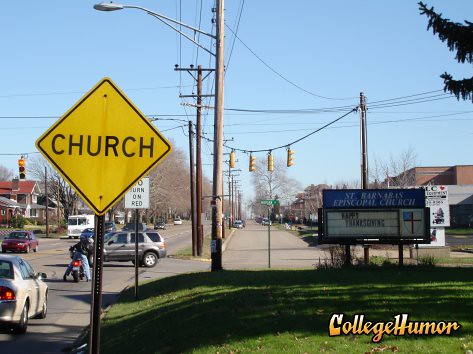The image depicts a busy street scene under a clear, blue sky. On the left side, there is a bustling road with several cars and a motorcycle, framed by houses with red, triangular roofs in the background. Prominently in the left foreground stands a yellow diamond-shaped sign on a gray metal pole, displaying the word "Church" in black text. The scene is intersected by another parallel street, with a cross street creating a junction controlled by a stoplight featuring four yellow lights hanging from wires. The right side of the image showcases a well-manicured lawn stretching to the street's edge and a sign for "Saint Barbara's Episcopal Church," adorned with a message wishing a "Happy Thanksgiving" in bold letters. Numerous electrical poles and black wires interlace the scene, enhancing the urban ambiance. Additionally, a small part of a tree is visible in the top right corner, adding a touch of greenery. The bottom right corner of the image features "College Humor" written in orange text. Overall, this detailed panorama captures the dynamic essence of a sunny day in a residential neighborhood.